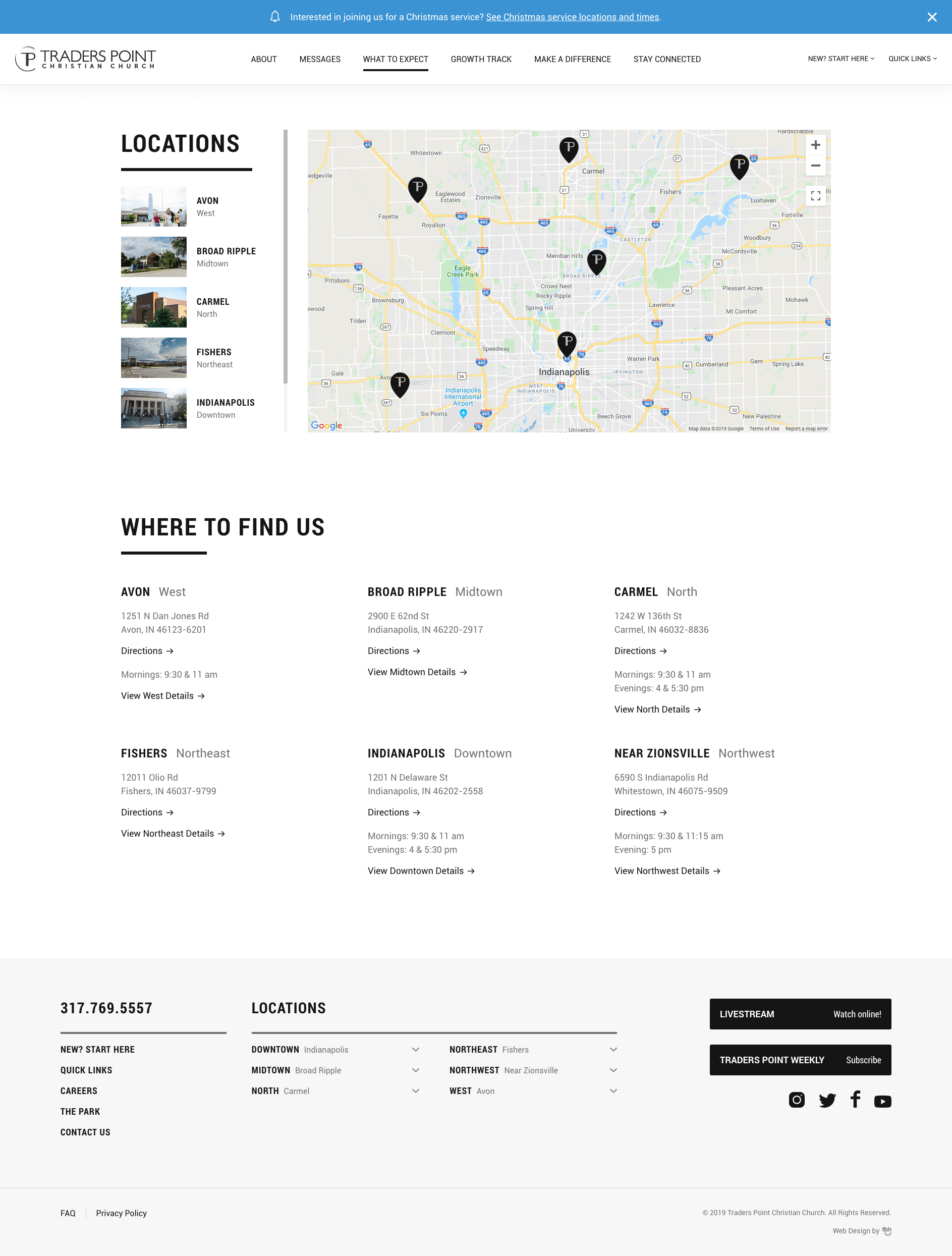The image displays a web page for Traders Point Christian Church. Near the top left corner is the church's name. Above it, a blue horizontal strip spans the top of the image, featuring white text that reads, "Interested in joining us for Christian service?" with an accompanying link stating, "See Christian service locations and times."

On the same line as the church's name and logo are several menu options: About, Messages, What to Expect, Growth Track, Make a Difference, Stay Connected, New Here, Start Here, and Quick Links. Below these options, a Google map is displayed, showing six locations of Traders Point Christian Churches, identifiable by the "P" in their location icons. The map centers around Indianapolis.

To the left of the map is a column featuring five pictures of specific locations, labeled "Locations." The images represent Downtown Indianapolis, Carmel, Broad Ripple, Avon, and Fishers.

Beneath the map and pictures is a section headed "This is where to find us," presented in black letters on a white background. It includes six addresses with links to directions for each location.